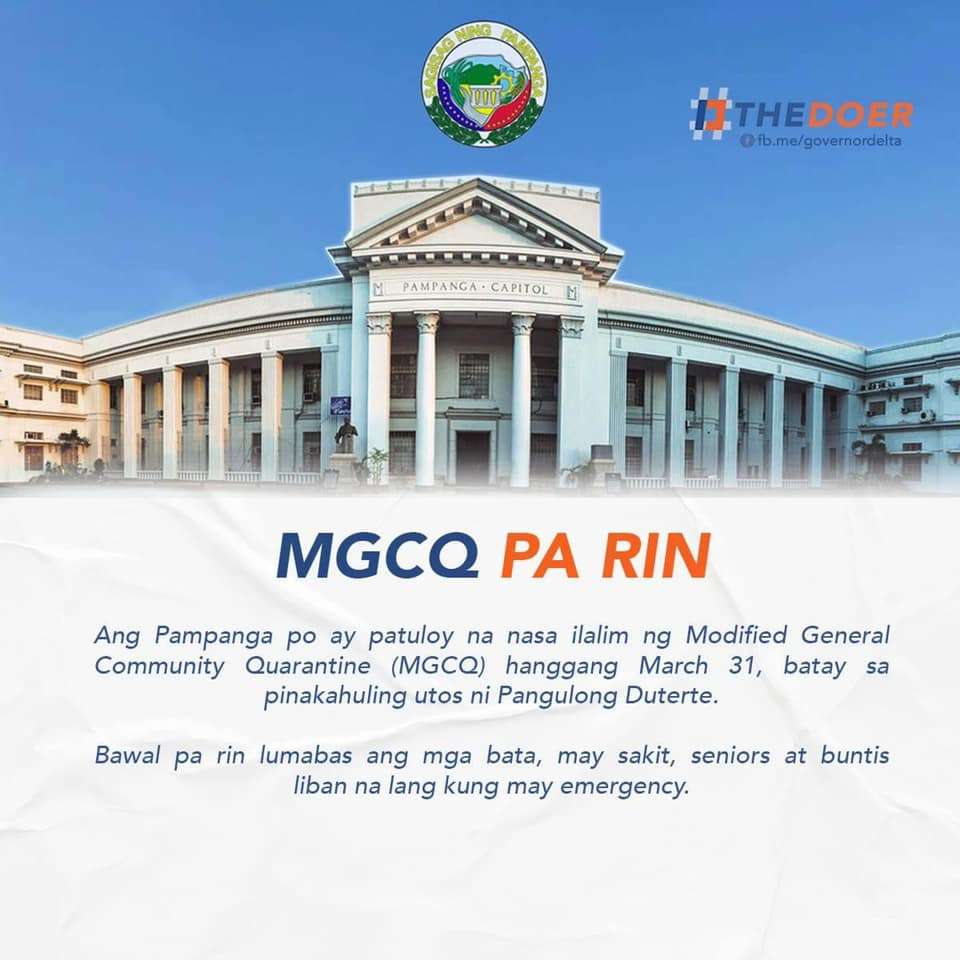The image is a flyer advertising a significant building, prominently featuring a large, white, government-style structure reminiscent of the White House. This imposing edifice bears the inscription "Pampanga Capitol" across its façade, flanked by white columns that cast dark shadows. Above the building, a national insignia featuring yellow, green, red, and blue colors is prominently displayed against a clear blue sky. To the right of this insignia is the phrase "The Doer" in a mix of blue and orange letters, followed by a URL: fb.me/GovernorDelta. In front of the building, on the left side, stands a statue of a person. The bottom portion of the flyer, set against a white background with a texture resembling crumpled paper, contains additional text. The top line reads "MGCQ" in blue, followed by "PARIN" in orange, with several more lines of text beneath in a foreign language, possibly Filipino, written in a blue font.